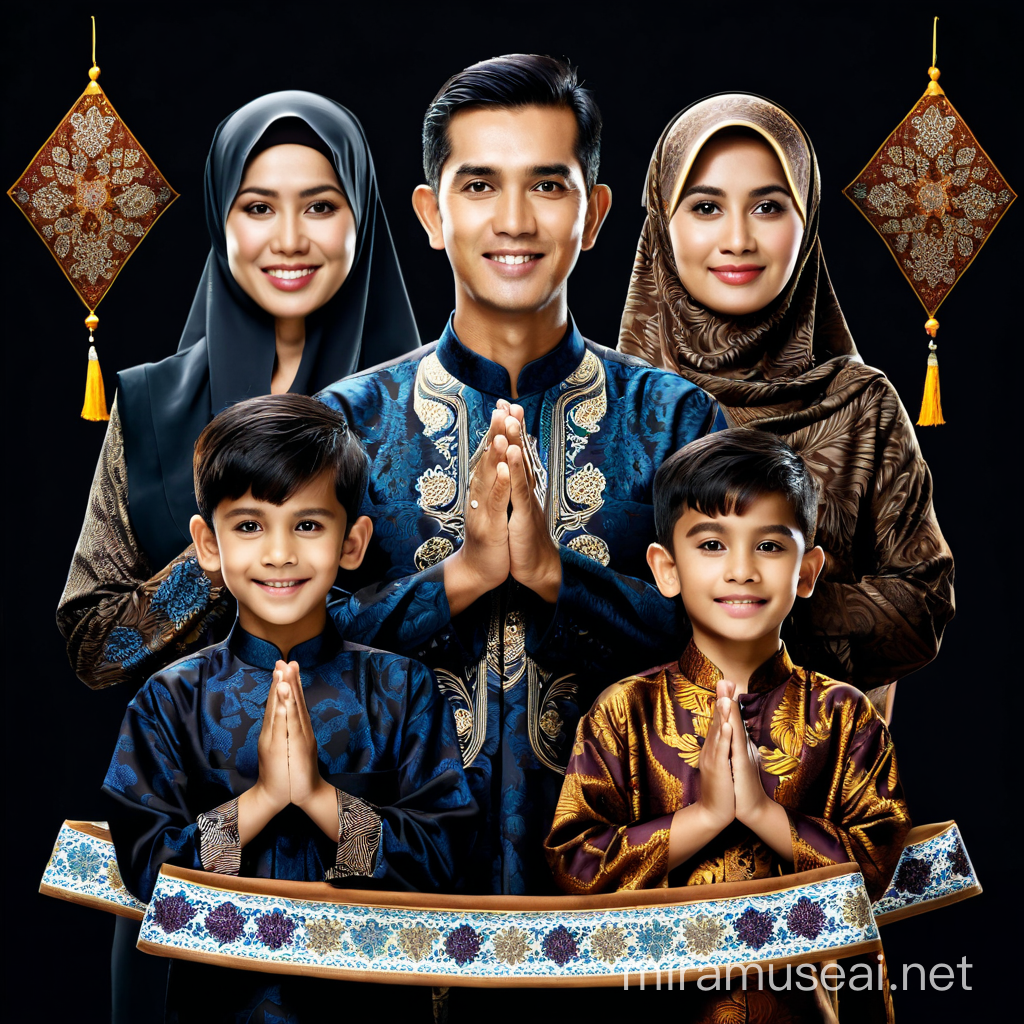This AI-generated family portrait depicts a South Asian family, possibly Indian, against a black background. At the center is a man in his 30s with short black hair, parted to the side, wearing a blue silk tunic adorned with a gold leaf pattern. His hands are folded in prayer, a gesture mirrored by the entire family, suggesting a religious context, possibly Muslim. Flanking him are two women of a similar age, both wearing headscarves; the woman on the left dons a blue headscarf and a red dress, while the woman on the right wears a brown headscarf with a brown dress. In front of the man are two young boys with parted dark hair, one in a blue tunic and the other in a gold-patterned tunic, both featuring intricate floral designs and golden tassels. Ornate, red diamond-shaped decorations hang from the ceiling with golden ropes in the upper corners. A blue and brown banner at the bottom, embellished with tan and white designs, completes the composition. All members of the family are smiling directly at the camera. The image is attributed to Mira Muse AI, indicating its digital creation.